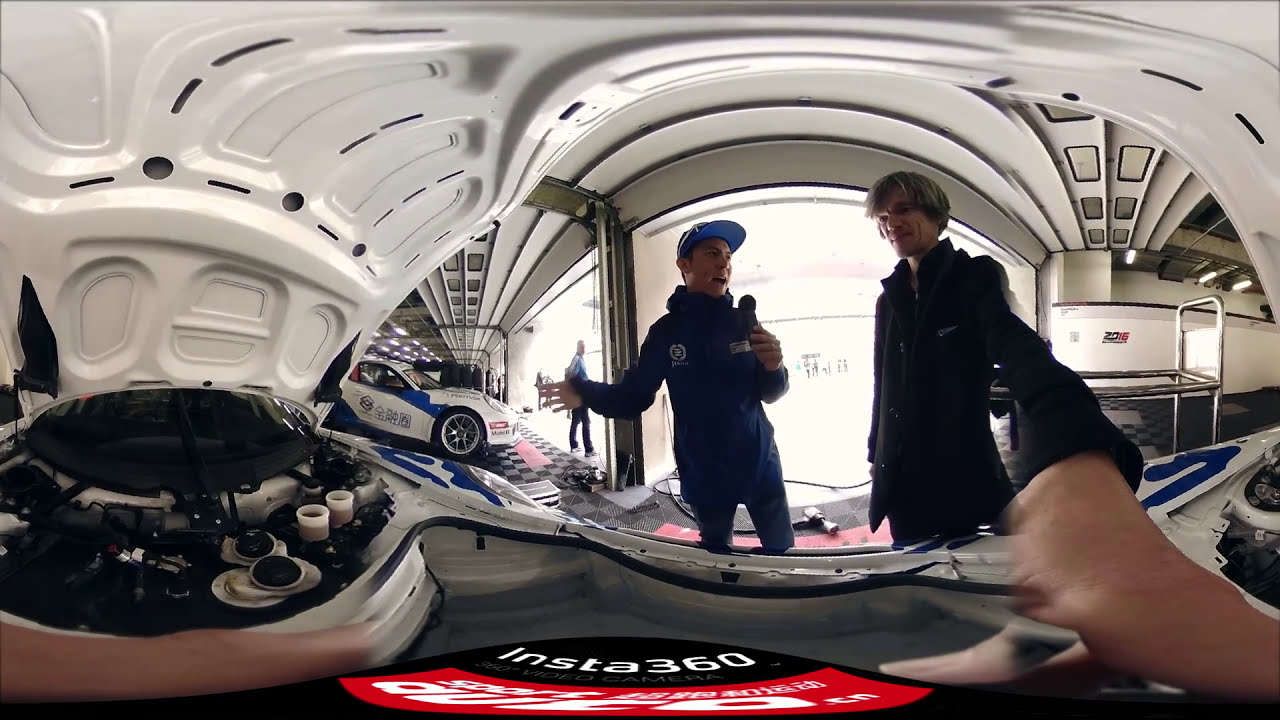This detailed panoramic image appears to be taken from the interior of a white, metallic, and plastic-looking compartment that resembles either an airplane or a spaceship, filled with various controls and indents potentially for storage compartments. The perspective is somewhat distorted, indicating it might have been taken with an Insta360 camera, which is partially visible at the bottom of the image.

In the center of the image, two men dressed in black bodysuits are looking towards the camera. The man on the left, who appears to be Asian and is wearing a blue baseball-style cap, seems to be holding a microphone. The man on the right, who has medium-length, blondish hair parted in the middle, extends his arm towards the camera, creating a blur that makes his hand appear exaggeratedly long.

Behind the men, on the left side, appears to be a race car with logos and blue trim, suggesting a fast, low-profile design. Close by, there’s a rack of tires and possibly a variety of pools. To the right, a metal cart can be seen behind the man extending his arm. Outside the bay window, another man stands in the distance, enhancing the scene’s depth. The overall image gives an impression of a high-tech, futuristic setting, possibly a movie set, with intriguing elements of both a garage bay and an advanced compartment interior.